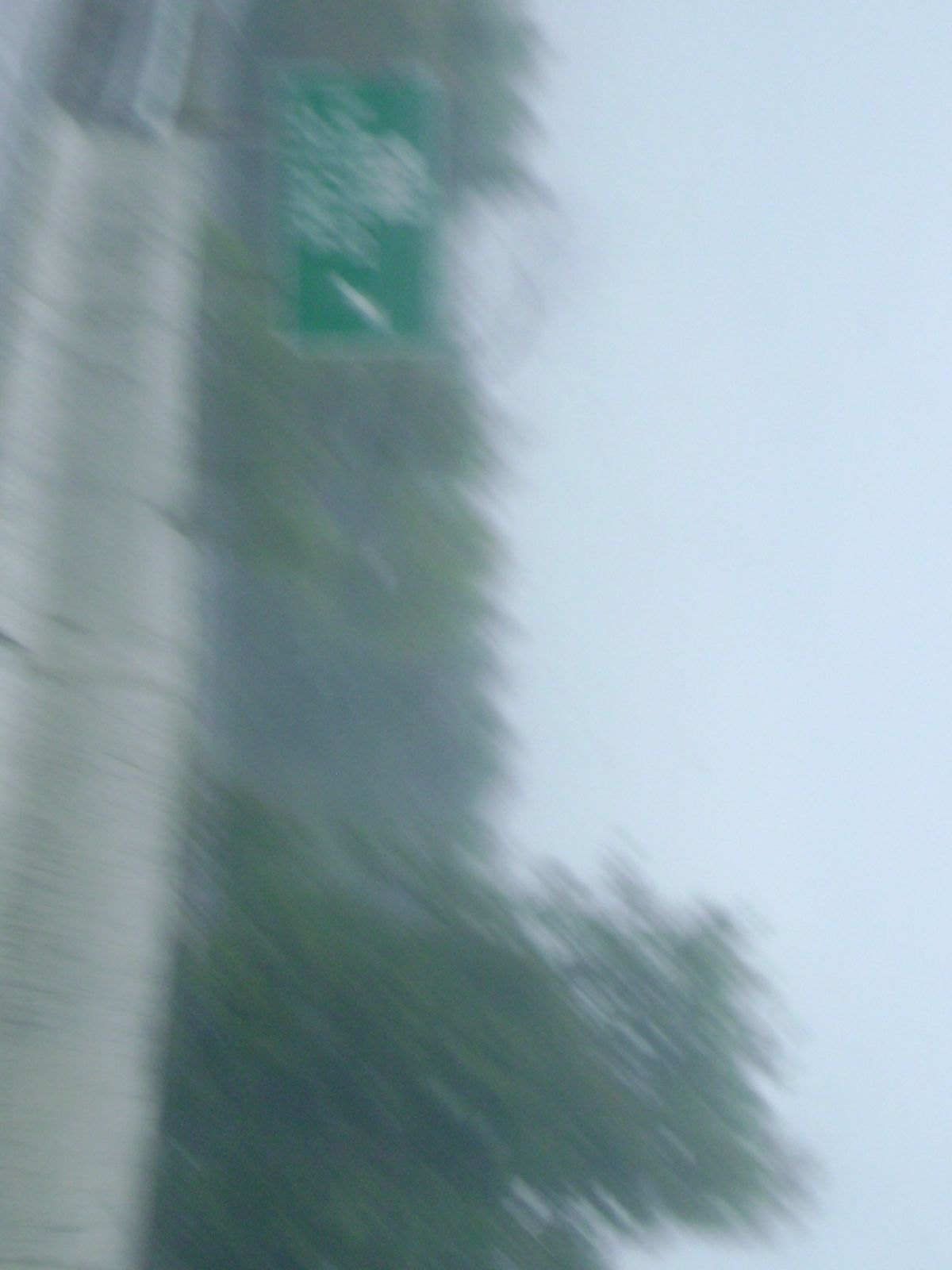This is a very blurry photograph, taken on a clear, sunny day and appears to be rotated 90 degrees, making the horizon vertical with the sky on the left. The image depicts a stretch of highway, with an off-white cement barrier running along the foreground. Beyond the barrier, a variety of trees dominate the scene, their details obscured by motion blur. In the top left section of the rotated image, there's a green highway sign with white lettering and an arrow, although the text on the sign is illegible due to the blur. The arrow is pointing towards what would be the right in the proper orientation. The clear sky is devoid of clouds, and a barely discernible vehicle can be seen towards the right, adding to the sense of motion in this dynamic yet unclear snapshot.